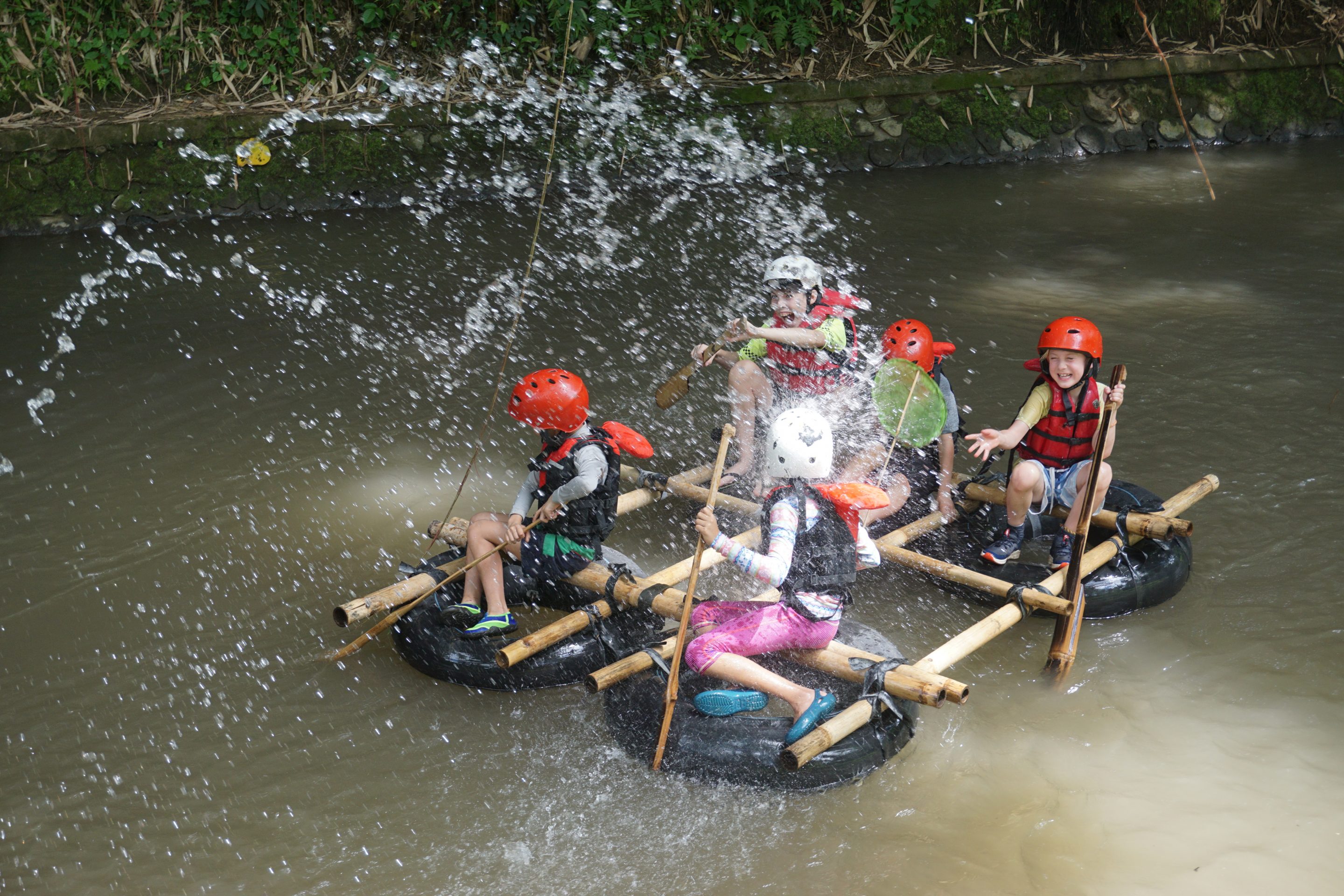This vibrant photo captures a joyful scene of five children on a makeshift raft navigating a shallow, murky creek surrounded by greenery and stones along the banks. The raft, ingeniously constructed from five black inner tubes, supports a lattice of hollow wooden poles tied together with black rope. Each child, smiling and laughing, sits on one of the poles. They use sticks as makeshift oars to paddle and splash water around. The children are well-equipped with safety gear: three wear orange helmets, while the two in the foreground sport white helmets. These resourceful adventurers appear to be thoroughly enjoying their playful and adventurous river tubing experience.